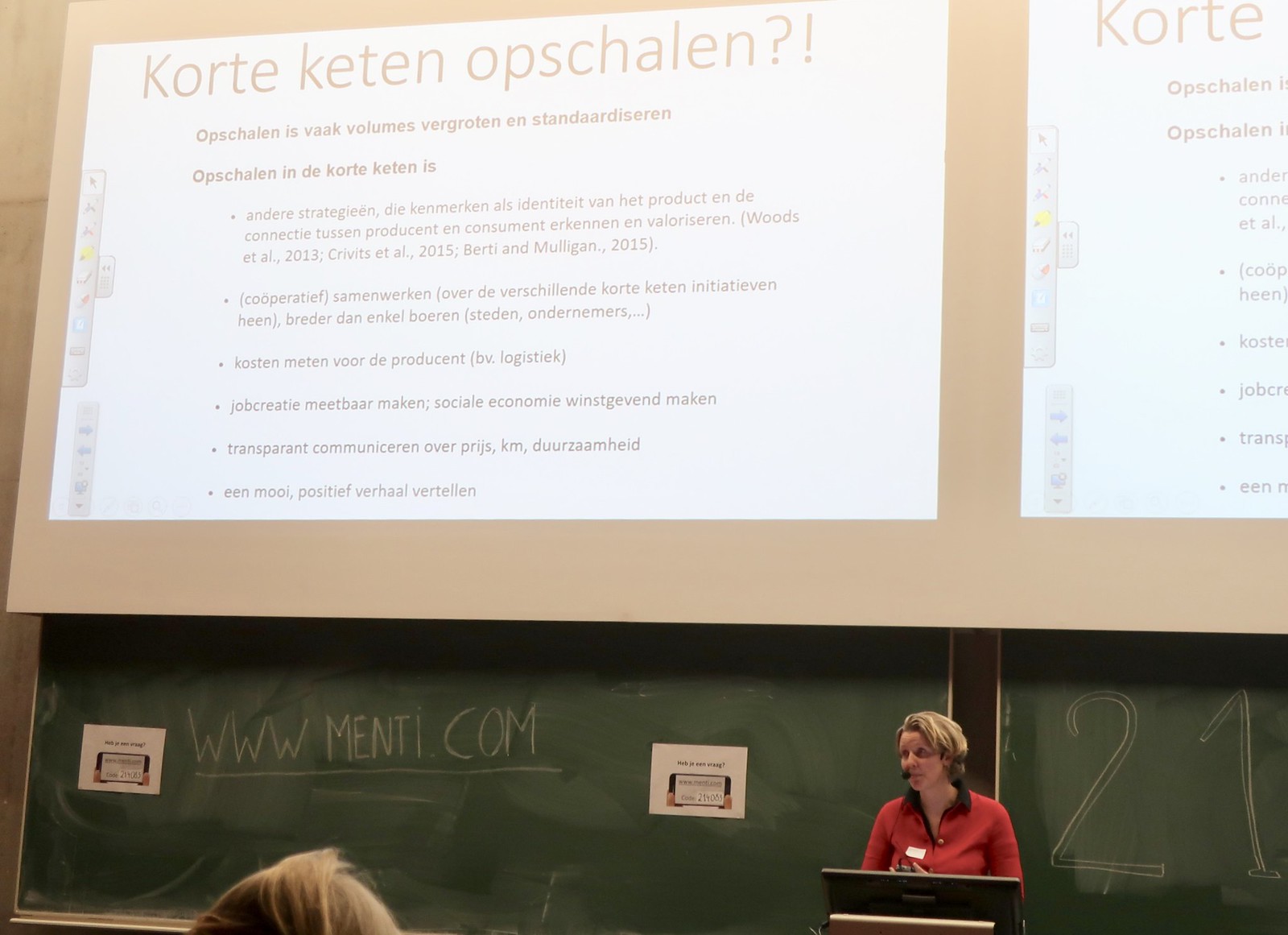This indoor photograph captures a woman presenting or teaching a class, characterized by a series of repeated visual elements and written text. At the lower center-right, the woman, wearing a red long-sleeve polo shirt with a black collar, stands at a podium with a headset microphone positioned by her mouth. She has short blonde hair and her head is turned slightly to the left. In front of her is the back of a computer monitor, suggesting she's using it for her presentation. The background features two green blackboards; the one on the right displays the number "21" while the board on the left reads "www.menti.com." There are a couple of pieces of paper posted on the signboards, but their content is illegible. Above her, projected onto a beige screen, the same document appears twice, both in white rectangles featuring text in a non-English language. The heading of the document reads "K-O-R-T-E, K-E-T-E-N, O-P-S-C-H-A-L-E-N?!" followed by a bullet-point list, suggesting it's part of a slideshow or presentation, possibly opened in a photo editor on her computer.